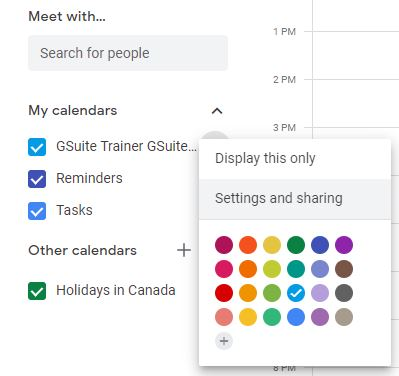This image depicts a close-up screenshot of a digital planner or task manager interface. The background is predominantly white, providing a clean canvas for the interface elements. 

In the top left corner, there is a small search bar labeled "Search for people." Directly below this, a calendar section features three blue checkboxes aligned vertically. Each checkbox is associated with a different category: "G-suite trainer," "Reminders," and "Tasks."

In the bottom right corner, a small pop-up window displays a palette of various color shades. This palette consists of numerous small, individually colored circles. The colors range from yellow, blue, purple, light gray, light purple, to red. Notably, there is a checkmark on one of the light blue circles, indicating it is selected.

At the top right side of the interface, time slots are listed vertically, showing 1 PM, 2 PM, and 3 PM, suggesting scheduled tasks or appointments during these hours. The overall design is organized and facilitates efficient task management and scheduling.